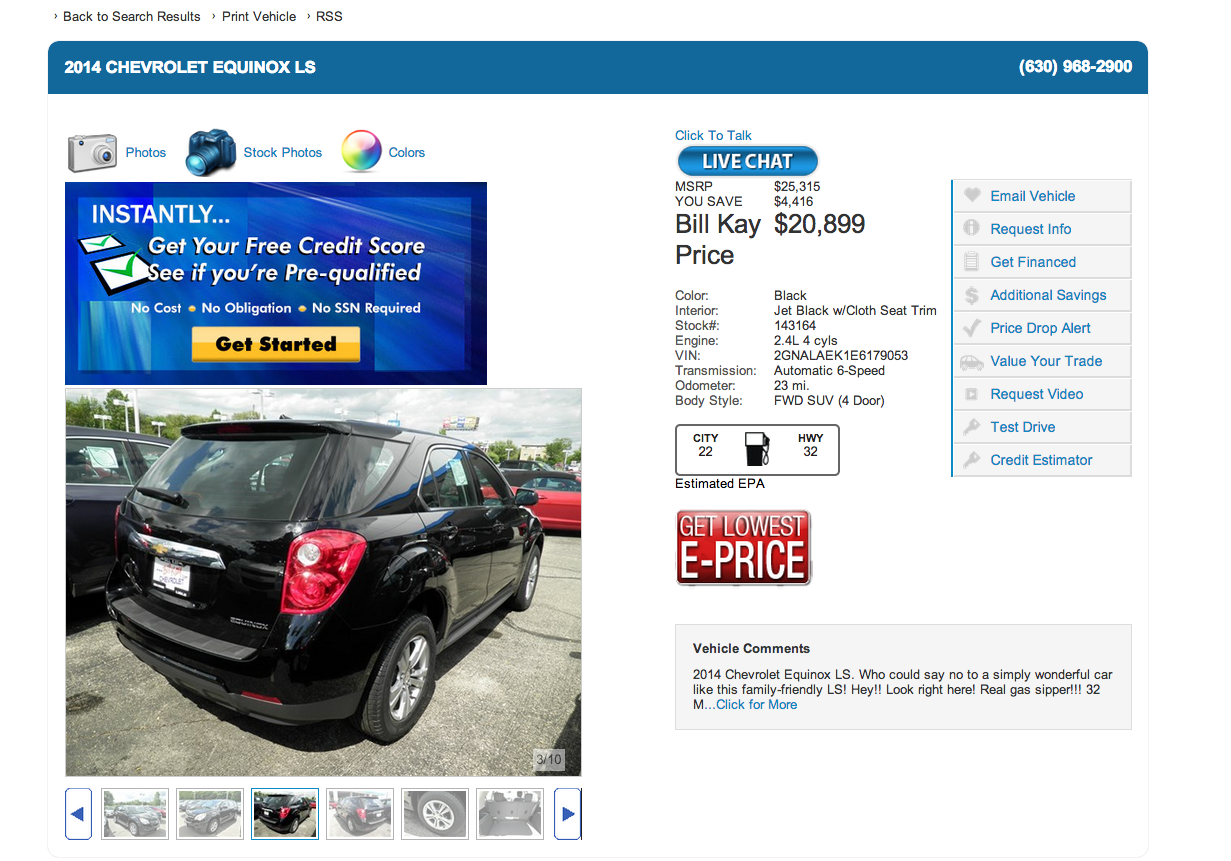In this webpage snapshot, a car listing webpage is displayed, featuring the details of a 2014 Chevrolet Equinox LS.

- **Top Right Corner:** The contact number for the dealership or website is prominently displayed as "630-968-2900."

- **Top Left Corner:** A navigation section is visible in black text, including options such as "Back to Search Results," "Print Vehicle," and "RSS."

- **Main Heading:** The model of the vehicle, "2014 Chevrolet Equinox LS," is clearly stated below the navigation.

- **Photo Categories:** Under the vehicle model, three categories are listed: "Photos," "Stock Photos," and "Colors."

- **Credit Information Section:** A blue box promotes a financial service with the message "Instantly... get your free credit score, see if you're pre-qualified. No cost, no obligation, no SSN required," followed by a "Get Started" button.

- **Vehicle Image and Navigation:** At the bottom left, there is an actual photograph of the vehicle, which is described as a black van with black wheels and red headlights. Navigation arrows on either side of the photo allow users to switch between images.

- **Price Information:** On the right side, a bold red square highlights, "Get Lowest Price," alongside the name "Billy K." The current price of $20,899 is displayed, compared to the previous price of $25,315.

This detailed breakdown provides a comprehensive view of the webpage and emphasizes the key informational elements for potential buyers.